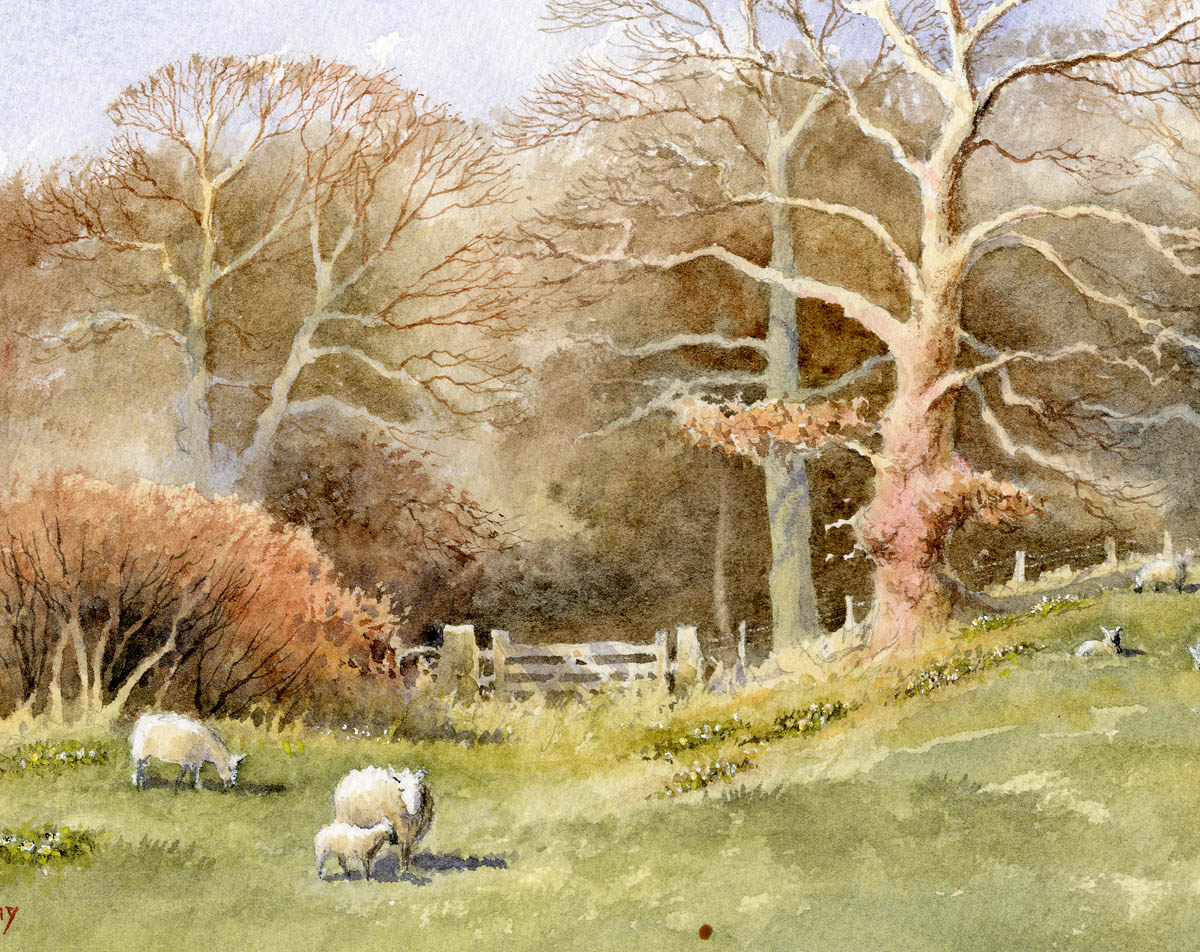The painting depicts a serene daytime outdoor farm scene in a nearly square format, focusing on a green, grassy pasture enclosed by a white gate in the lower center. The sky, a soft blue occasionally dotted with clouds, dominates the upper left portion, with trees lining both the left and right sides. These trees vary: some are bare, revealing the turning of seasons with hints of fall colors, while others display sparse leaves in shades of orange and brown. Sprinkled throughout the green pasture are several sheep, grazing peacefully. On the lower left, three sheep stand together, one of which appears to be a young lamb. Towards the right, another lamb lies down, with a few more sheep scattered around—a mix of standing and reclining figures. The grass is depicted in varied hues of green, dotted with occasional flowers, contributing to the pastoral charm. The scene evokes a tranquil farm life, emphasizing the harmony between nature and its inhabitants.